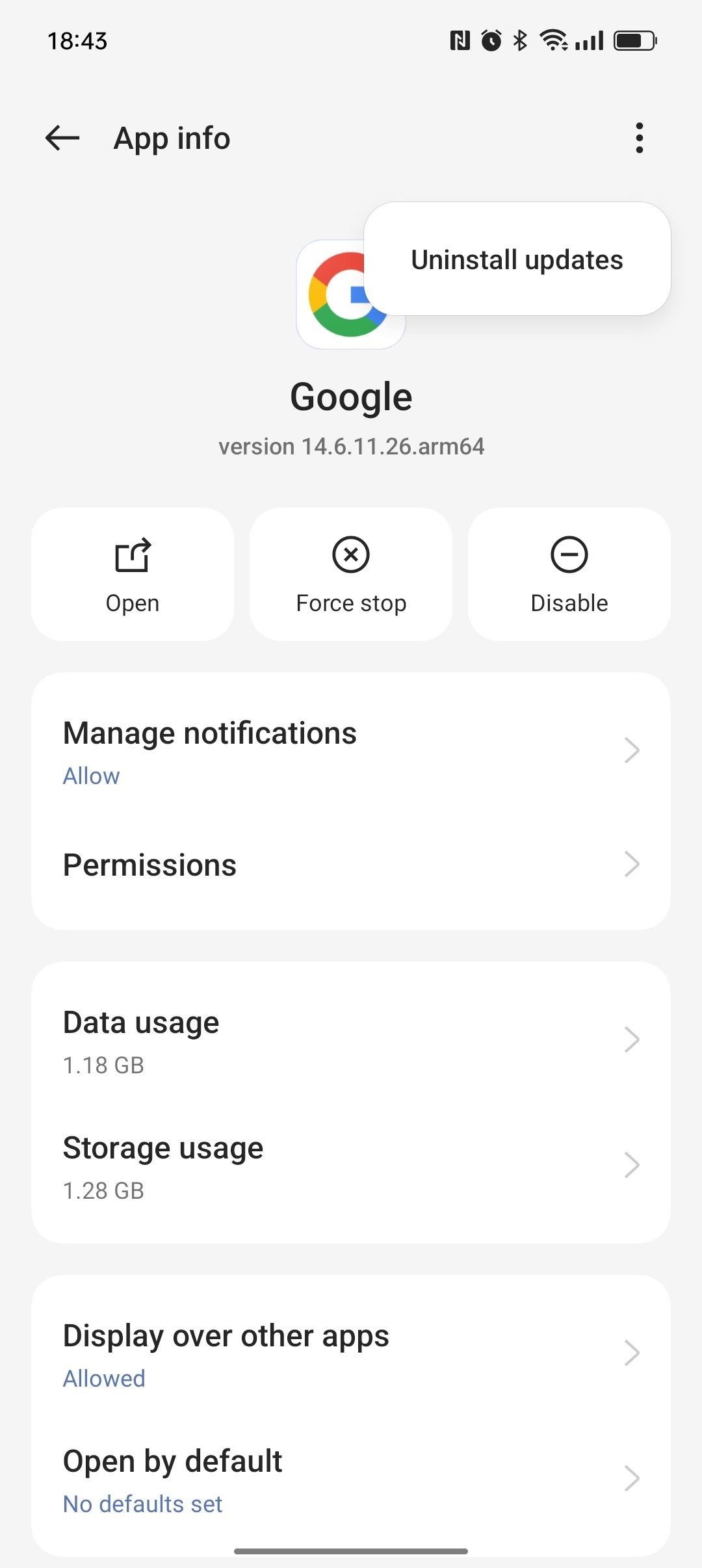This is a detailed screenshot taken from an Android phone, showcasing the settings for the Google app. The battery indicator in the upper right corner shows approximately 75% charge, and the time displayed to its left reads 18:43 (6:43 PM). At the very top of the screenshot, "App Info" is prominently displayed with a leftward pointing arrow beside it, indicating a navigation option. On the right-hand side, the three-button menu icon is visible, which, when tapped, reveals a drop-down menu. This has been activated, showing the "Uninstall Updates" option.

In the middle of the screen, the Google logo is prominently displayed with "Google" written beneath it. Just below, the app version is listed as "14.6.11.26 ARM64." Three buttons appear below this version information: "Open" on the left, "Force Stop" in the middle, and "Disable" on the right.

Further down, various app options are detailed. The "Manage Notifications" option is set to "Allow." The "Permissions" section is shown, followed by "Data Usage," which accounts for 1.8 GB. "Storage Usage" is listed as 1.28 GB. At the very bottom, additional settings are indicated: "Display Over Other Apps" is marked as "Allowed," while "Open by Default" shows "No Default Set."